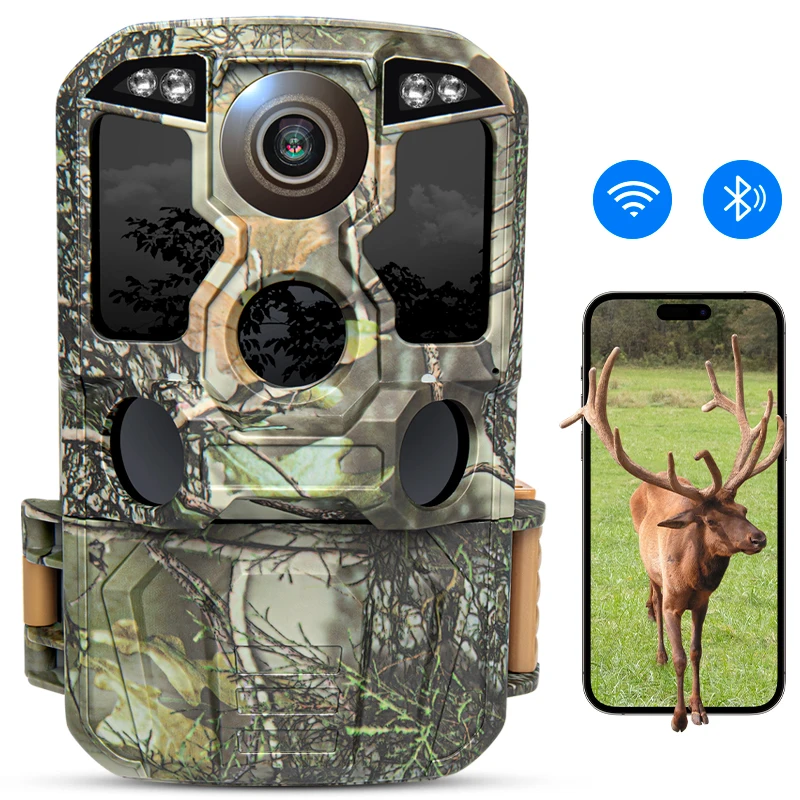The image features a unique, camouflaged case that appears to be designed for a camera or a high-tech device. The case, which has a rugged and sturdy appearance with its mix of grays, whites, and hints of green, has a circular cutout in the center, likely for a camera lens, along with two reflective or mirror-like circles on either side resembling windows. The background is white, providing a stark contrast to the detailed case. On the left side of the image, there's an illustration of a cell phone with a similar camouflage pattern, where the camera sits at the top center with two lights flanking it, and small icons indicating sound and Bluetooth functionality. On the right side, an iPhone screen displays a vivid scene of a forest with grass, featuring a moose prominently in the foreground. Interestingly, the moose appears to extend beyond the phone's screen, suggesting a layered or augmented reality effect. The combination of detailed case design and the lifelike forest scene creates an intriguing juxtaposition that hints at both rugged outdoor usage and advanced technological features.